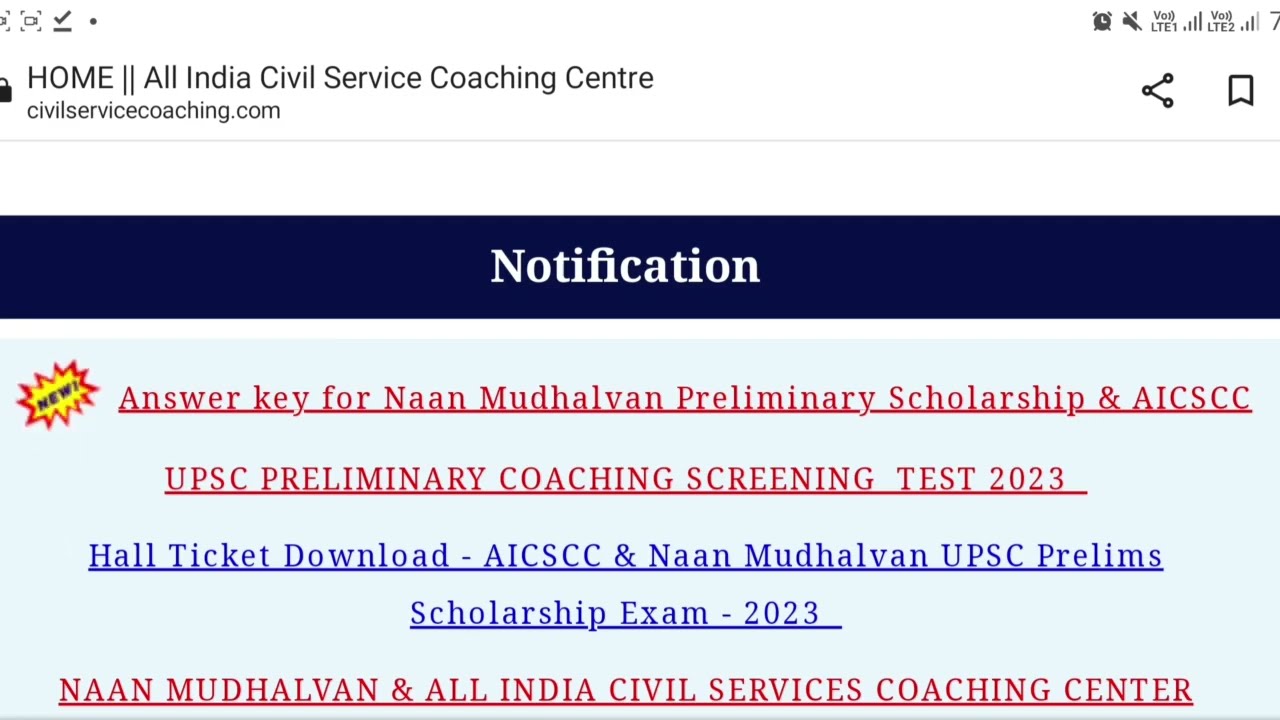The screenshot appears to be taken from a mobile device, evident from the phone symbols in the upper right corner. The top of the screen contains text that says "Home All India Civil Service Coaching Center" and the website "CivilServiceCoaching.com". Below this header, there is a prominent section labeled "Notification." In this section, there are various links and messages. The most notable link, highlighted in red, reads "Answer Key for Non-Mudhalvan Preliminary Scholarship in AICSCC." Another link, also in red, states "UPSC Preliminary Coaching Screening Test 2023." Additionally, a blue-colored link offers a "Hall Ticket Download" for the AICSCC and Non-Mudhalvan UPSC Prelims Scholarship Exam 2023. The colors used in the screenshot include yellow, red, dark blue, light blue, medium blue, white, and black. The overall style and structure strongly indicate that it is a mobile screenshot, confirmed by the presence of a share button and a bookmark symbol in the top right.